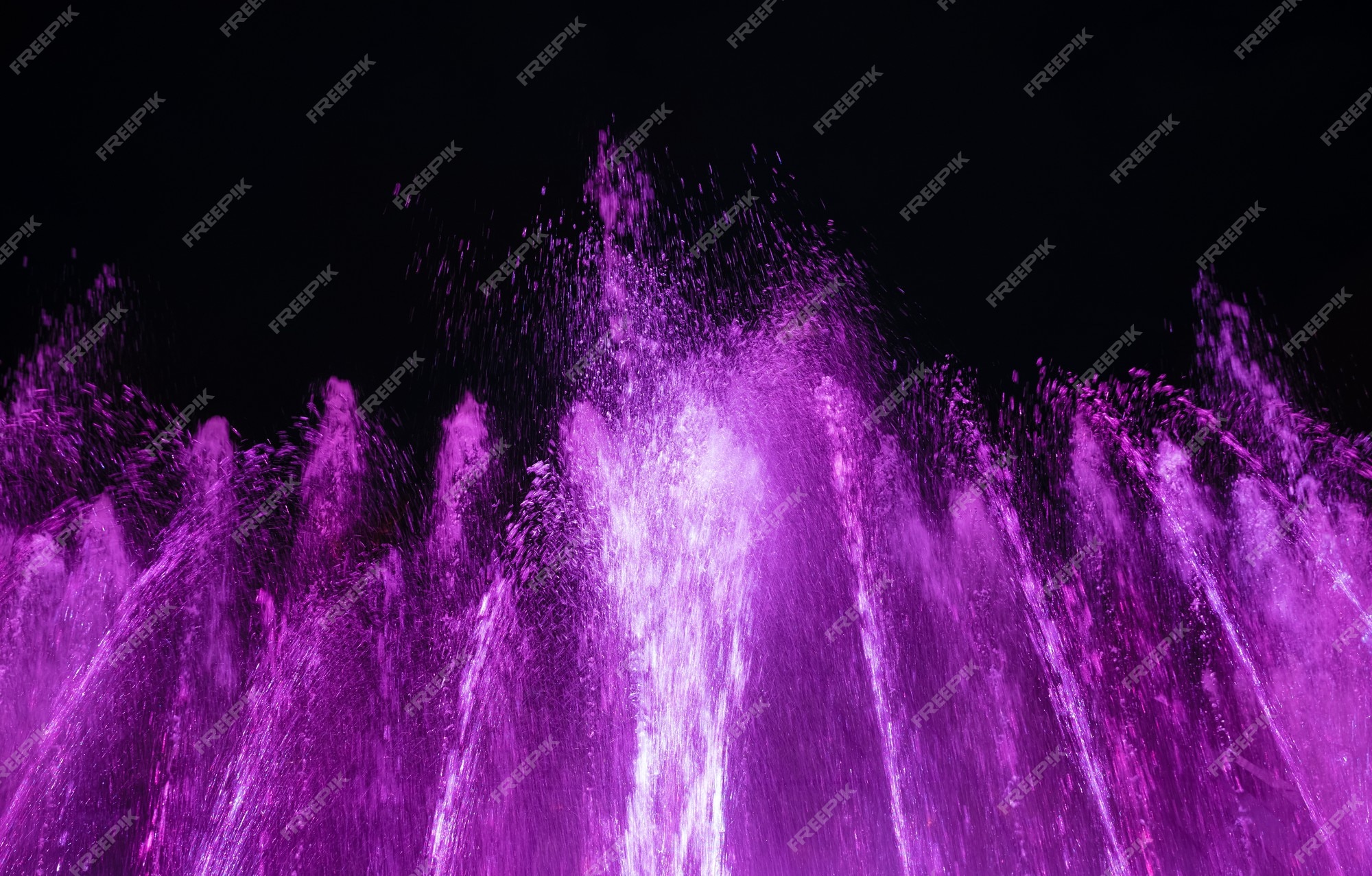The image depicts what appears to be a photograph of a large, elaborate fountain, reminiscent of the water show at the Bellagio in Las Vegas. Set against a night sky that is pitch black, the fountain’s numerous jets of water shoot upwards in graceful arcs. These jets are lit with a stunning gradient of magenta, purple, and pink hues, with the tallest central jet displaying a mix of white light, illuminating the scene dramatically. Above the geysers, droplets of water linger in the air, adding to the sense of movement and fluidity. A noticeable watermark reading "freepik" stretches across the entire image, arranged in multiple diagonal rows from the top left to the bottom right corner, indicating the image’s protected status.